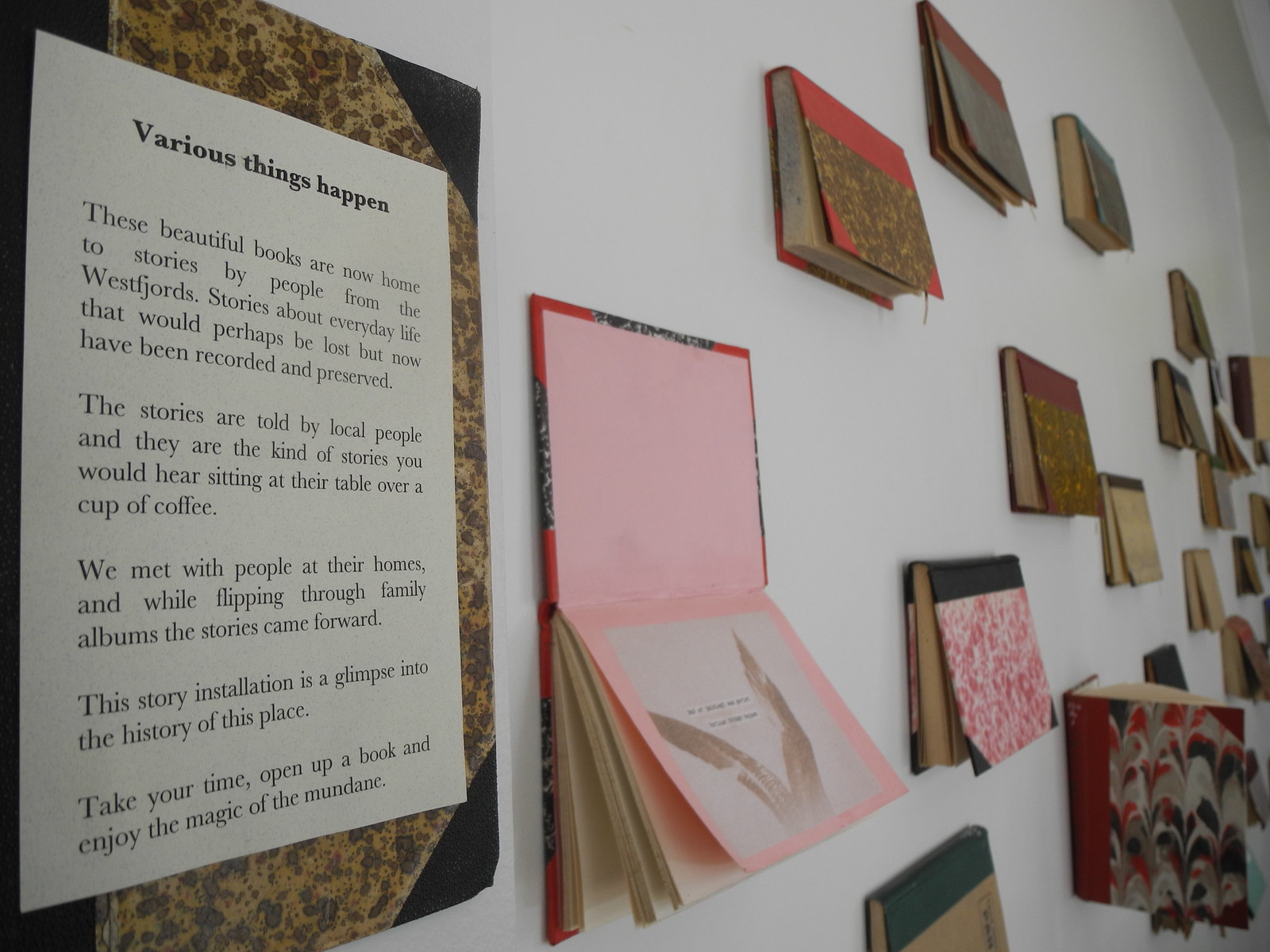The image captures a compelling museum exhibit found within an art gallery, comprising numerous hardcover books mounted onto a white wall. These books have been stripped of their jackets and are affixed to the wall by either their front or back covers, allowing visitors to flip through them. Each book carries its own unique, colorful binding. Prominently displayed next to the installation is a placard that reads, "Various things happen. These beautiful books are now home to stories by people from the West Fjords. Stories about everyday life that would perhaps be lost but now have been recorded and preserved." These stories, recounted by local people, evoke the intimate, anecdotal narratives one might hear while sitting at a table over a cup of coffee. The creators of this exhibit met with locals in their homes, and as they flipped through family albums, these stories emerged. This immersive installation offers a glimpse into the rich history of the West Fjords community. Visitors are encouraged to take their time, open up a book, and indulge in the magic of the mundane. Along the wall, the books are thoughtfully arranged—some open horizontally with their pages cascading downwards, others closed, but all are filled with personal stories waiting to be discovered.